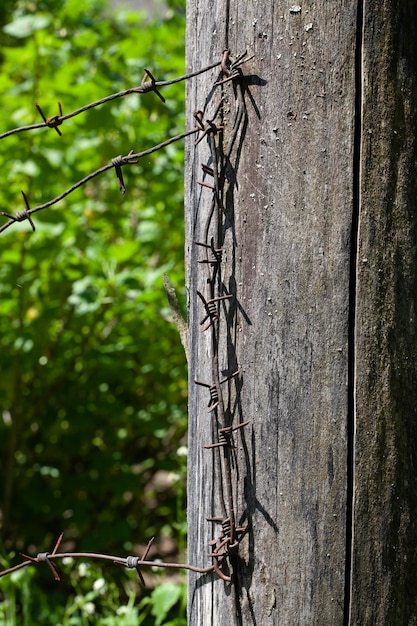The image depicts a weathered wooden post positioned on the right side, adorned with dark gray, rusted barbed wire that extends towards the left. The wooden post exhibits signs of aging with visible cracks and a mix of grays and dark tans, hinting at prolonged exposure to the elements. Numerous metal spikes and remnants of past attachments are embedded in the post. On the left side, bright, vibrant green leaves bathed in sunlight provide a vivid contrast to the muted tones of the post and wire. The image, which is oriented as a vertical rectangle, captures a rustic scene with a mix of natural and man-made elements, possibly situated in a residential area.